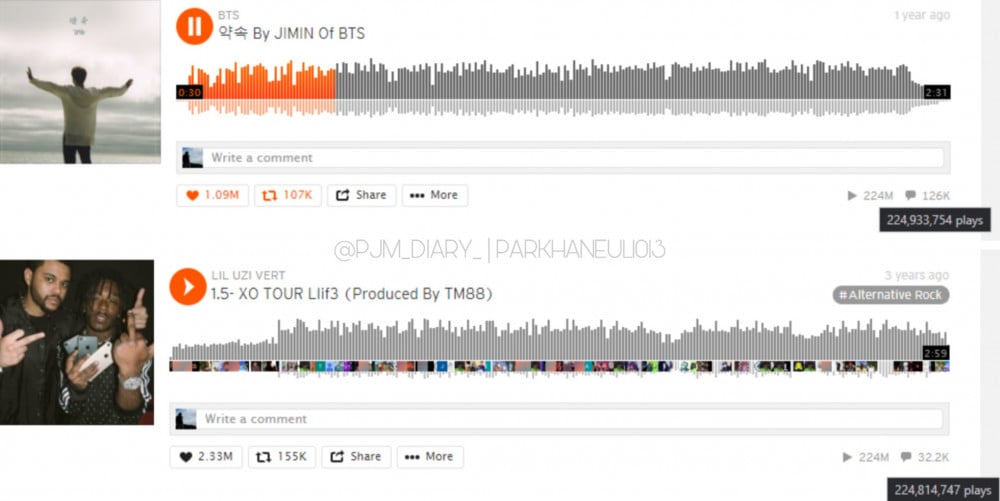This image is a screenshot from SoundCloud, showcasing two different songs in the playlist. 

The first song at the top displays its cover image, featuring a person dressed in a long white sweater, posed with arms outstretched, resembling a T-pose. Above this image, the text reads "BTS" followed by a string of Korean characters, indicating that the song is performed by Jimin of BTS. The song's progress bar is partially filled with an orange color, indicating that the track is currently being played.

The second song listed below is a collaboration between The Weeknd and Lil Uzi Vert. At the top of this entry, "Lil Uzi Vert" is prominently displayed, followed by the song title "1.5XO to our life", indicating the track's unique name and artistic partnership.